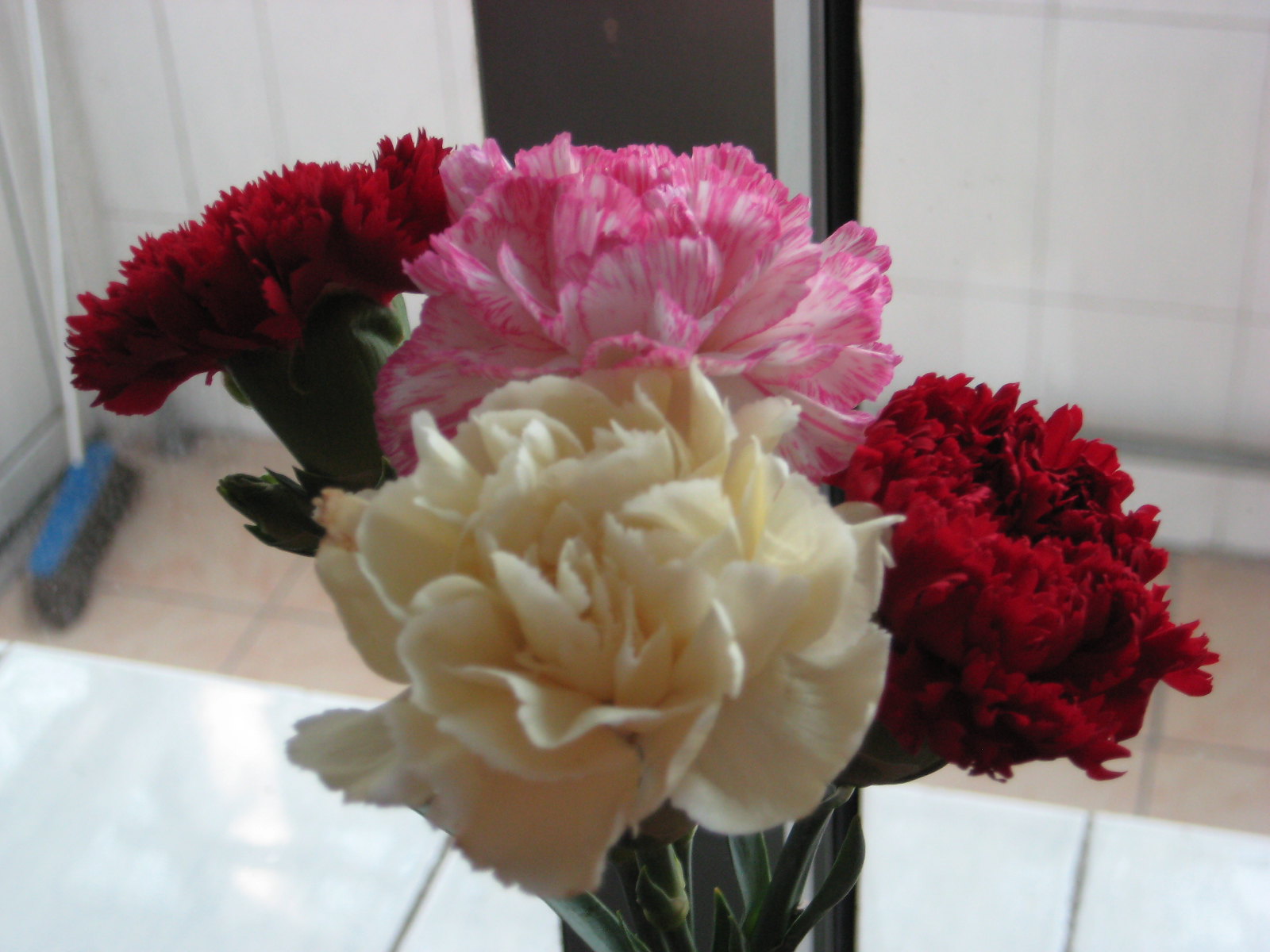The image is set indoors and depicts a close-up of a vase with four carnations positioned on a white, tiled countertop. The visible portion of the white vase is adorned with a green leaf pattern. Among the flowers, a pristine white carnation is placed prominently at the forefront. Just behind it and slightly elevated is a pink carnation with white petals tipped in medium pink hues. To the left, slightly higher and turned towards the back, sits a dark red carnation, and to the right and slightly lower, another deep red carnation is visible. The stems and greenery are noticeable beneath the flowers. In the background, cabinetry, a white wall, and a beige tiled floor are visible. A blue push broom with a white handle leans against the left side of the wall, adding a touch of everyday domesticity to the scene.